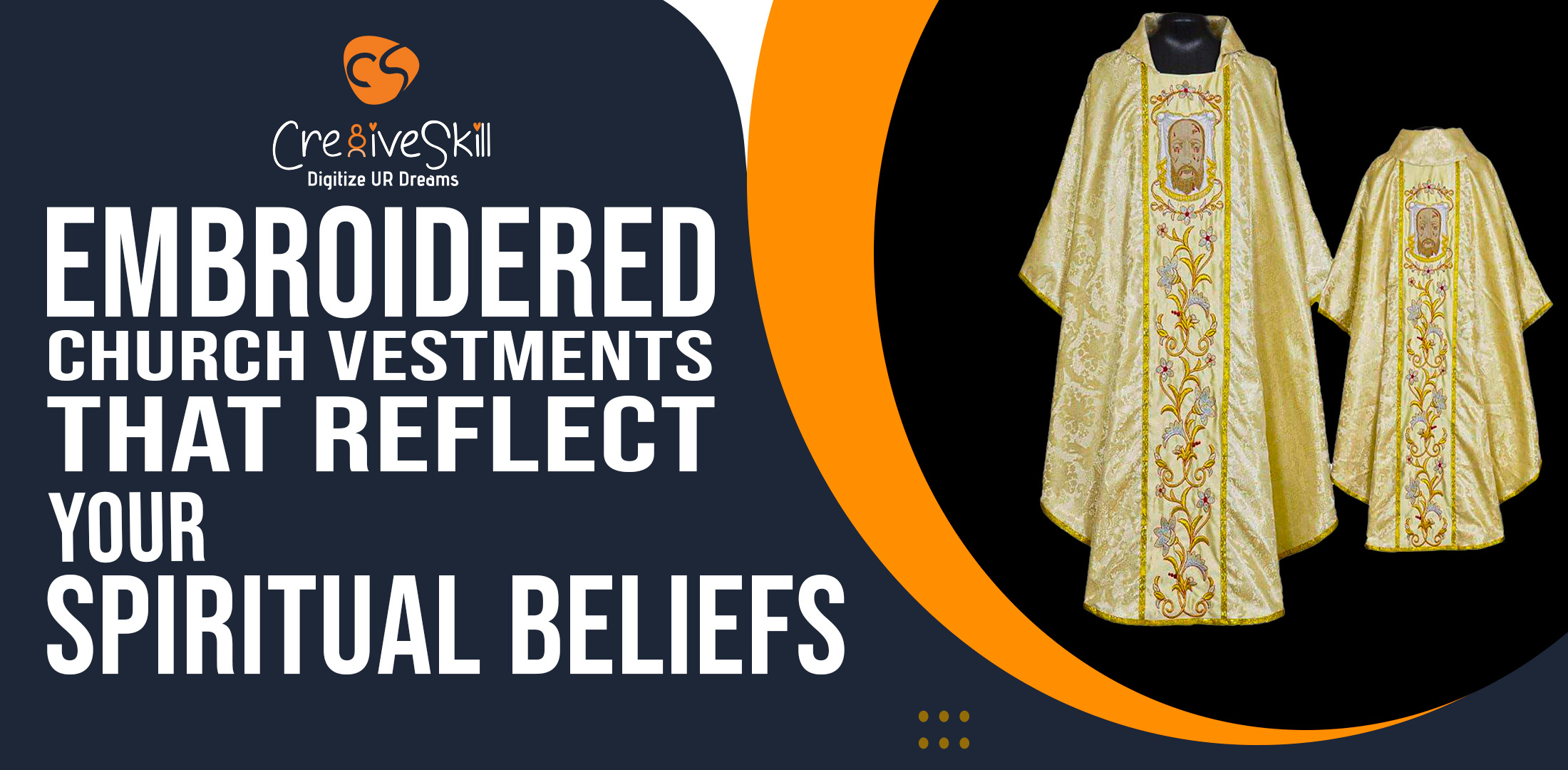The advertisement is rectangular and features a dark gray background. Dominating the left side, in bold white letters, is the tagline: "Embroidered Church Vestments that Reflect Your Spiritual Beliefs." Below this, the Creative Skill logo—a C and an S within an orange circle resembling a rounded triangle—appears, accompanied by the phrase "digitize your dreams" written in white lowercase letters.

On the right side of the advertisement, an orange swoop flows from the top to the bottom. This swoop encircles a black area which prominently displays two gold religious robes, adorned with intricate embroidery. Each robe features a central image of a man's face on the chest, surrounded by blue floral and gold vine accents. The robe on the left appears larger and closer, while the one on the right appears smaller and further in the distance. Towards the bottom right, there's a decorative element comprising three orange circles aligned vertically, both at the top and the bottom, forming a rectangular pattern.